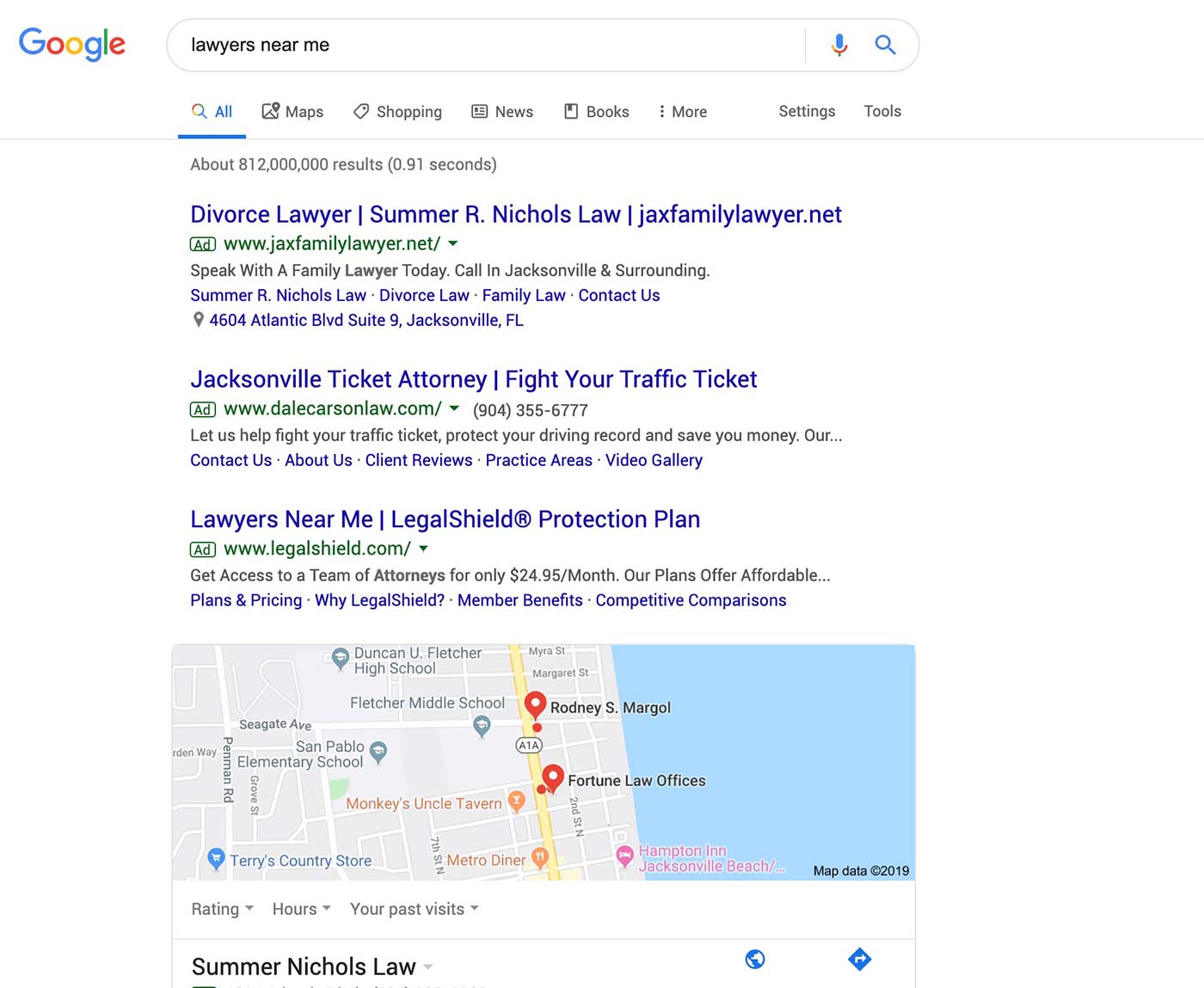A vertical image displays a Google search results page on a white background. At the top-left corner, the traditional Google logo in its vibrant colors is prominently visible, followed by a search bar with the query "lawyers near me" entered. Adjacent to the search bar are the microphone and magnifying glass icons. Below the search bar, an array of clickable options are displayed, with "All" selected and highlighted in blue. Other options available include Maps, Shopping, News, Books, More, Settings, and Tools. 

The page details the number of search results and the time taken to generate them. Further down, several specific search results are listed. The first result features "Divorce Lawyers, Summit R. Nichols Law," accompanied by its web address, a brief description, and contact information, including the physical address. The next listing highlights "Jacksonville Ticket Attorneys," with details on fighting traffic tickets, including a phone number, web address, and additional links for contact, about us, client reviews, practice areas, and a video gallery. Another result, "Lawyers Near Me, Legal Shared Protection Plan," comes with a brief explanatory blurb. 

At the bottom, a map showcases the locations of these search results, with "Summit R. Nichols Law" prominently marked.